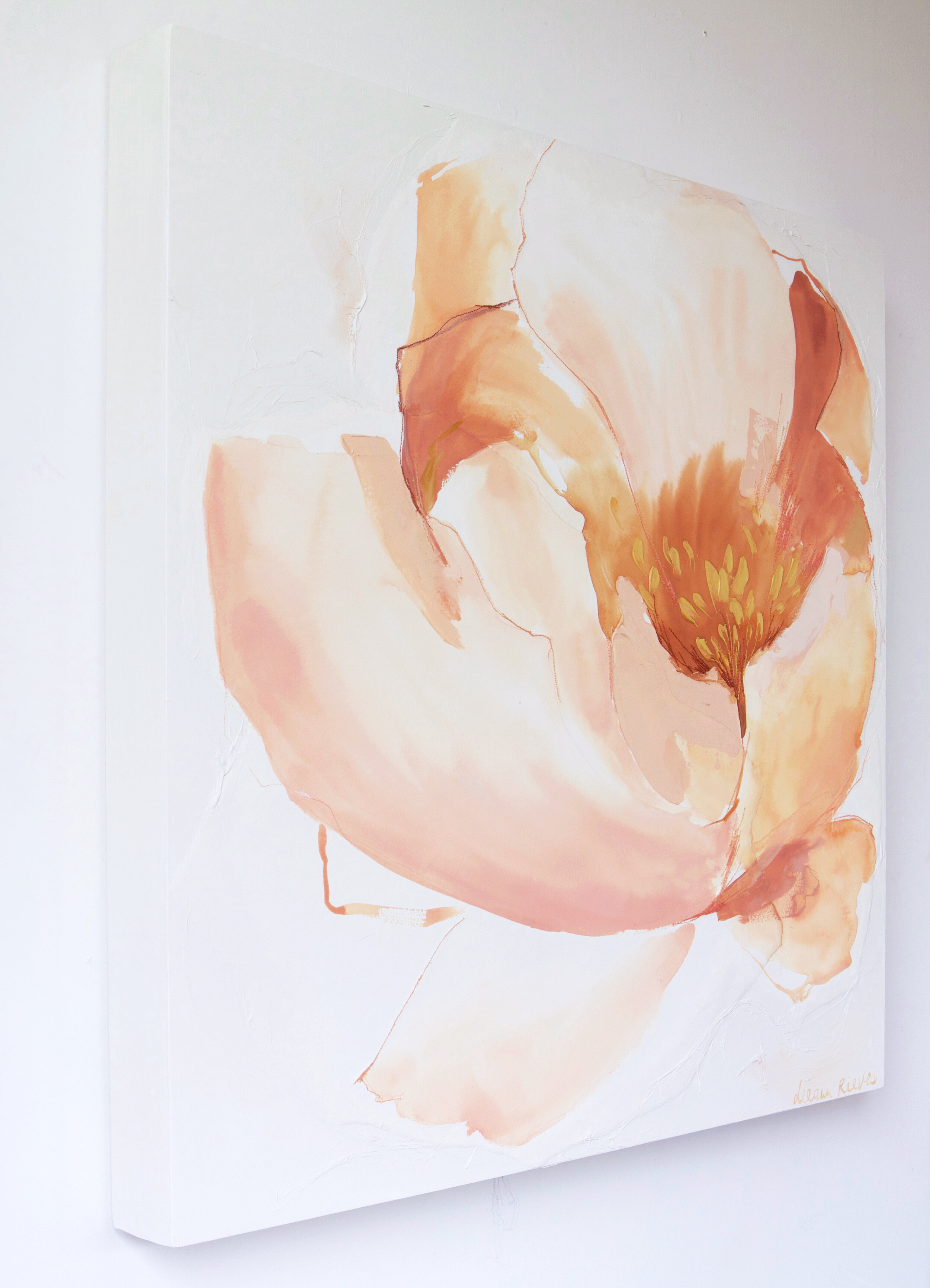The image depicts a highly detailed watercolor painting of a flower on a white canvas. The captivating artwork is prominently featured on an upright, frameless canvas, which is displayed against a white and gray background. The flower, characterized by its vibrant palette, consists predominantly of peach, orange, pink, and reddish-orange hues. The petals of the flower are gracefully splayed outwards and occupy nearly the entire canvas, leaving little empty space. Central to the bloom, the pistils are painted in rich orange and yellow tones, adding depth to the composition. The lighting in the image is bright and even, ensuring the painting’s intricate details and vivid colors are clearly visible.